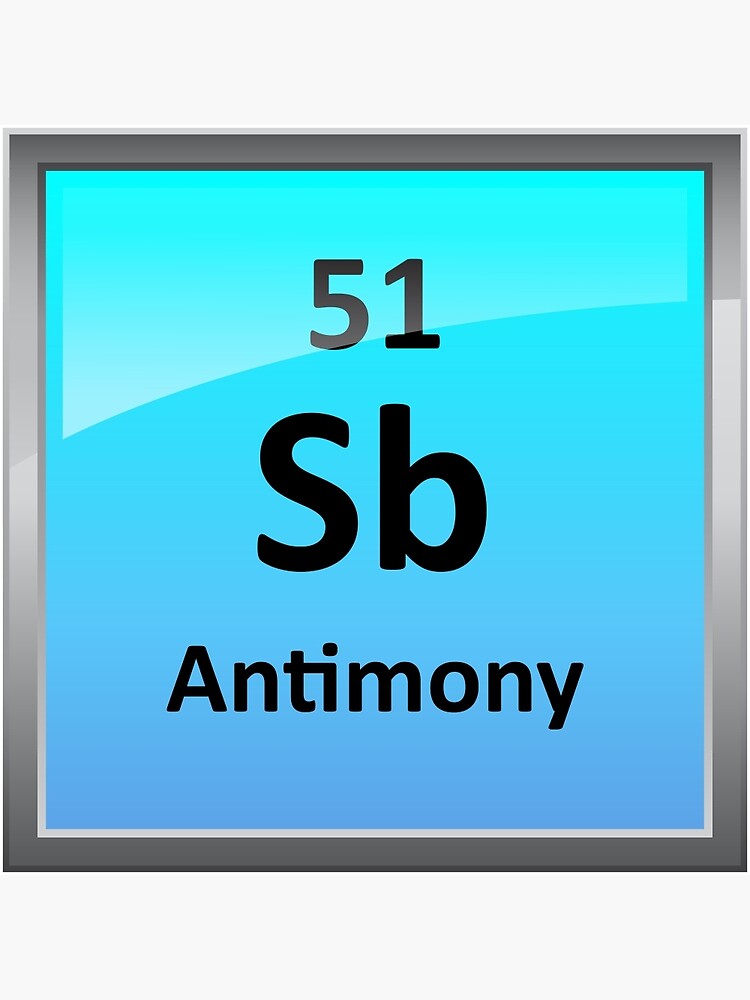This image is a digitally rendered icon resembling an element from the periodic table, housed in a square frame with a silverish-gray border. The background of the icon is primarily blue, with multiple gradients from light to dark. At the top, a lighter blue area with a reflective glare on the upper left corner gradually transitions into a slightly darker blue. Prominently displayed at the top in large black numerals is the atomic number "51." Below this, in bold black letters, are "Sb," with the "S" being capitalized and the "b" in lowercase. Further down, the background shifts to an even darker blue, where the element name "antimony" is written in black letters. This image, simple in design, features a basic 3D animation style reminiscent of Windows PixArt graphics.